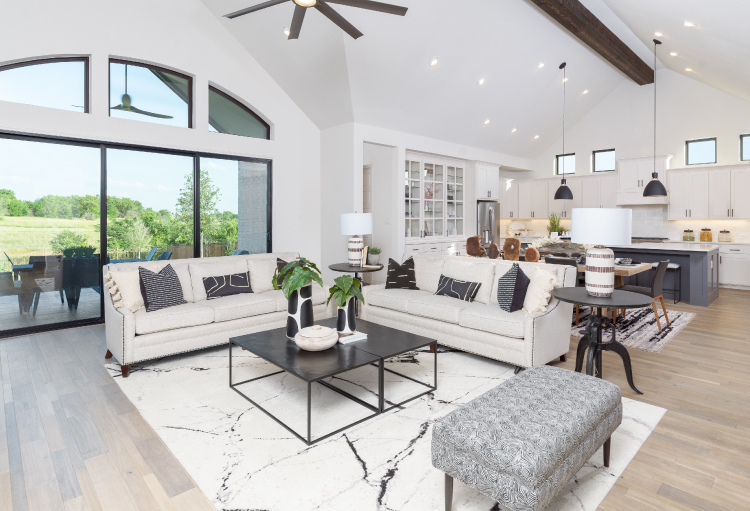This image showcases the interior of a spacious, modern home with an open living space design, boasting predominantly clean and white decor. The central focus is the living room, featuring two white couches adorned with gray and black pillows, a white and black marbleized area rug, and a gray marbleized ottoman. Dark brown side tables with lamps, and a striking black coffee table complete the chic setup. Overhead, a wooden ceiling fan adds a touch of warmth.

To the center right of the image lies a stylish kitchen, identifiable by its sleek, white cabinets and a gray island. The kitchen is illuminated by two low-hanging black pendant lights. The design seamlessly transitions from the living room to the kitchen, with an open layout enhancing the sense of spaciousness.

On the center left of the image, tall glass panes or sliding doors lead out to a patio, allowing natural light to flood the space and further highlighting the modern architecture of the home.